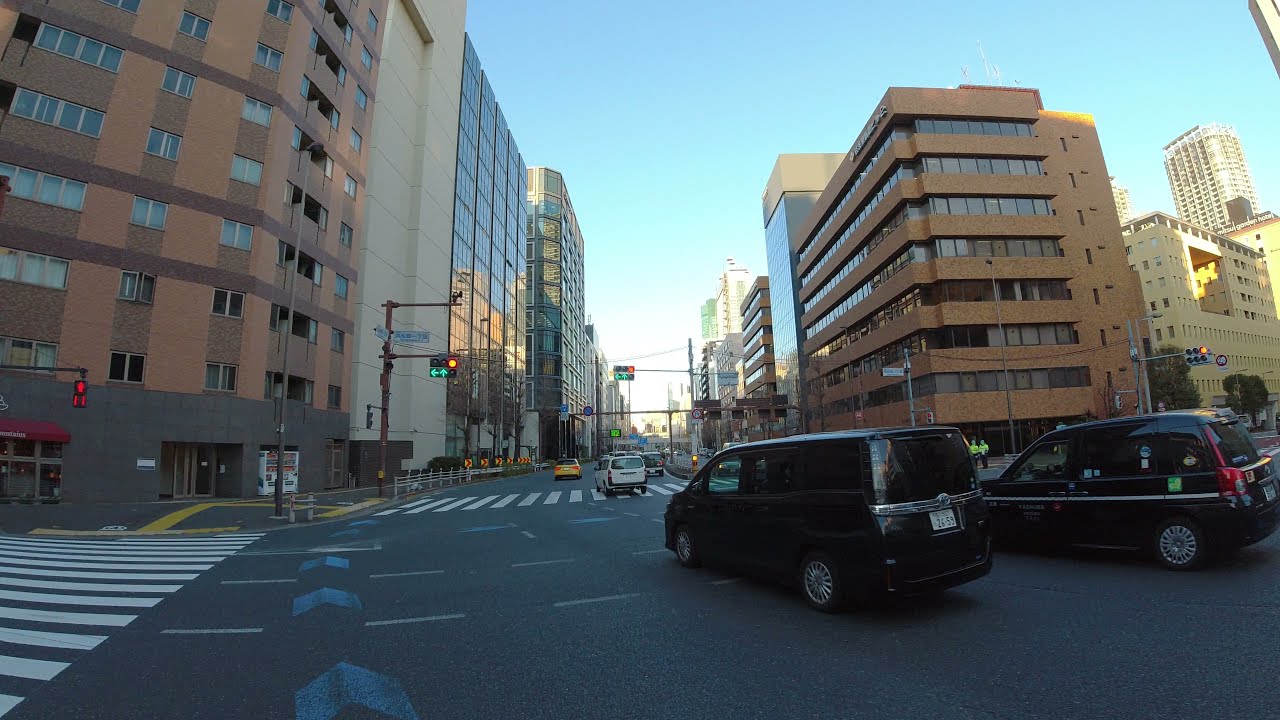This image is a color photograph in landscape orientation, capturing a bustling daytime city scene from a sidewalk at an intersection. Dominating both sides of the street are tall buildings with a mix of architectural styles—some with numerous glass windows, others of light brick, brownstone, and white stone. The sky above is a clear, vivid blue, adding a bright backdrop to the urban landscape.

In the foreground on the bottom left corner, we see a white pedestrian crosswalk leading to a light brick building. The intersection features traffic lights, with a visible street light showing a walk signal.

The street itself is busy with several cars. Prominently in the lower right corner, there are two black vehicles—a van on the left and a small car to its right. Further down the street, which recedes into the distance, are more cars, including what appears to be a white van and a yellow car, possibly a taxi. These vehicles populate the center of the image, adding to the dynamic, lively atmosphere of the city.